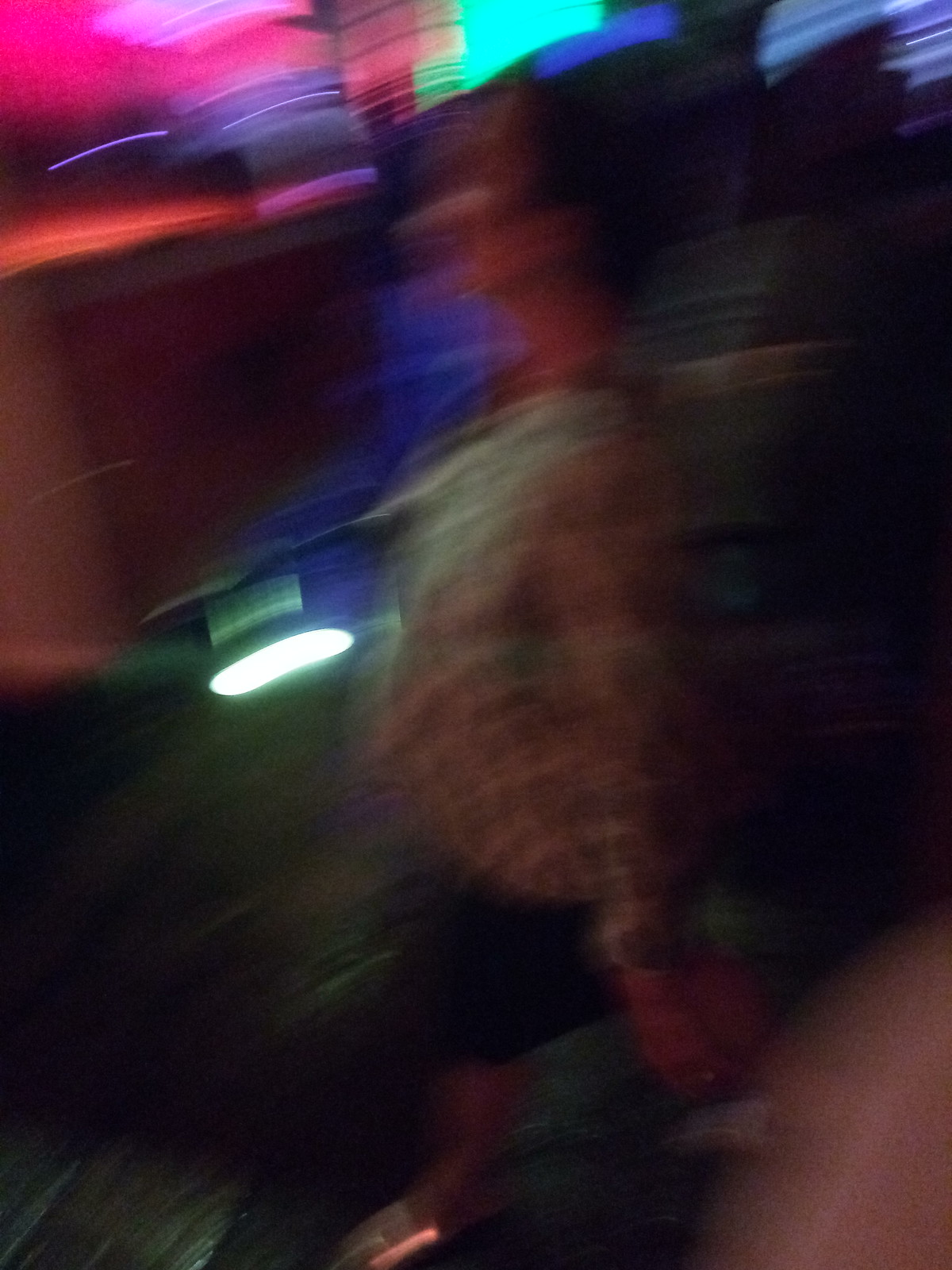A dimly lit, blurry photograph captures a human figure in motion, facing left, in either a poorly lit interior or a nighttime setting. The image is out of focus, with smears obscuring details, yet we can discern that the person is wearing a long-sleeved shirt and dark pants. Before the figure, a bright, oval-shaped light punctuates the scene. Above and ahead of them, vibrant streaks of colorful street or neon lights sporadically illuminate parts of their face and upper chest, creating a striking contrast against the dim background.